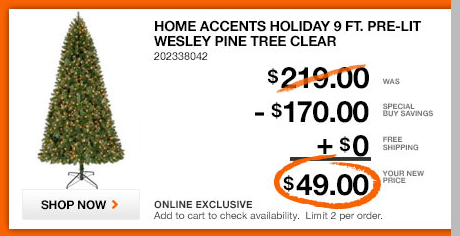**Advertisement Screenshot Description:**

This image appears to be a screenshot of an advertisement. It is structured in a horizontal rectangle format.

**Left Side:**
On the left side of the image, there is a depiction of an artificial Christmas tree. The tree is pre-lit and features a visible metal stand, indicating that it is designed for easy setup and stability.

**Right Side:**
- **Title:** The title of the product is prominently displayed in all capital letters: "Home Accents Holiday 9FT Pre-lit Wesley Pine Tree, Clear."
- **Product Code:** Below the title, a numeric product code is listed: "202338042."
- **Original Price:** Slightly to the right, the original price "$219" is displayed in large print, with a diagonal orange line striking it out.
- **Discount Information:** To the right, the text reads "was $219" and underneath, the discounted price of "$170" is mentioned along with the phrase "special buy savings."
- **Shipping Details:** Below the discount information, it states "Plus $0" and to the right, "free shipping."
- **Final Price:** There is a highlighted section showing the final price of the product, which is "$49." This price is circled in orange, giving it a hand-drawn marker appearance.
- **Additional Information:** To the right of the circled price, it states "your new price."
- **Online Exclusive:** Beneath the price details, it mentions "online exclusive."
- **Purchase Limitation:** At the bottom, there is a note stating "add your cart to check availability, limit two per order."

This detailed and visually engaging advertisement emphasizes the significant discount on the pre-lit Wesley Pine Christmas tree and includes essential product and purchasing information.